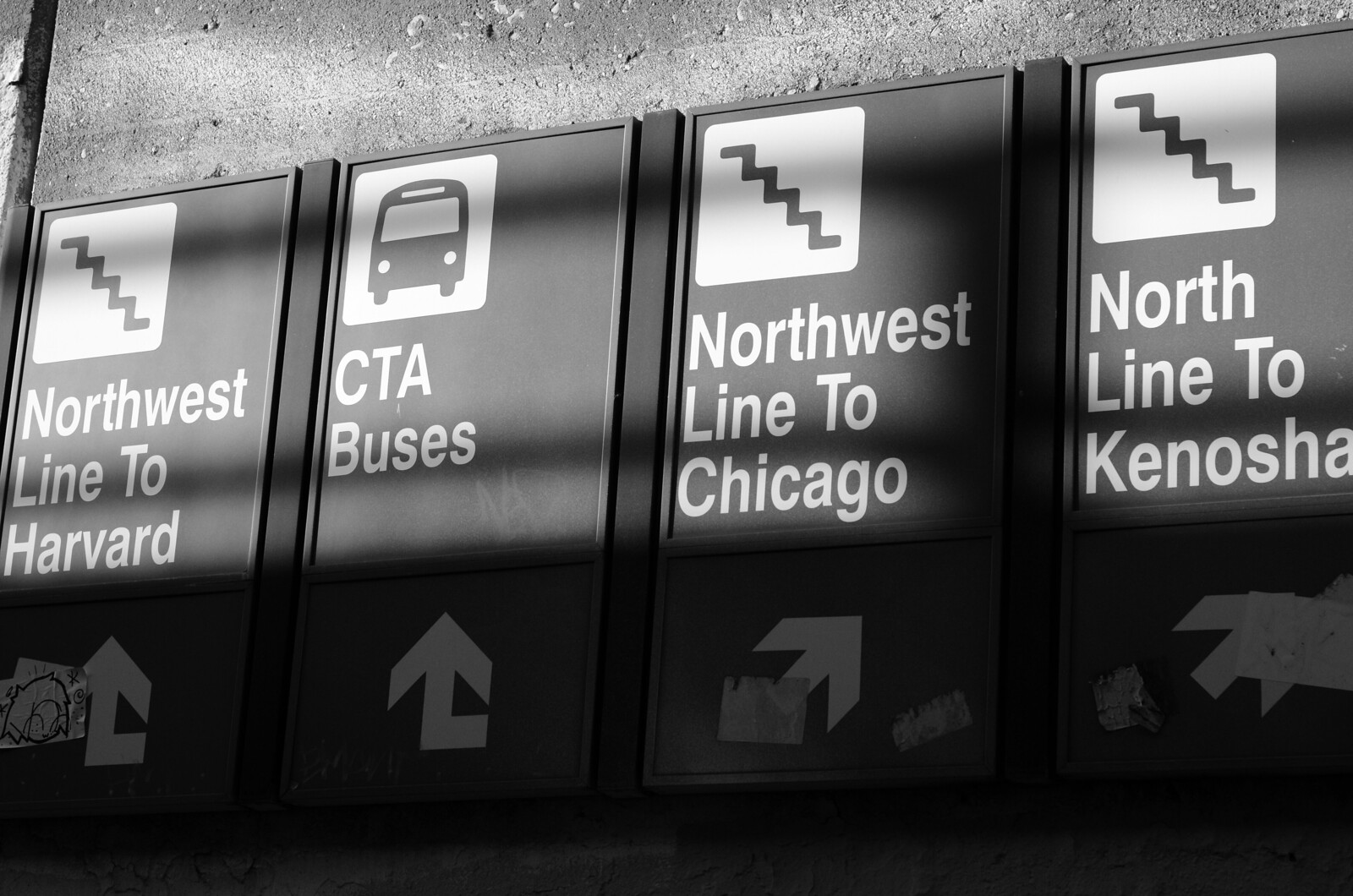In this modern black-and-white photograph, four directional signs are neatly arranged in a row on a solid cement wall, guiding travelers to different transit destinations within the city. The leftmost sign features an icon of stairs in a white box, with the words "Northwest Line to Harvard" in white font, accompanied by an upward-pointing arrow. Next to it, the second sign includes a simple black bus icon with the label "CTA buses," also directing travelers straight ahead. The third sign displays another set of stairs in a white box, indicating the "Northwest Line to Chicago," with an arrow pointing upwards and to the right. Lastly, the far-right sign features the same stair icon with the text "North Line to Kenosha," directing travelers with an arrow pointing to the right. These distinct yet cohesive signs efficiently convey directional information, helping pedestrians navigate their way through the transit system.